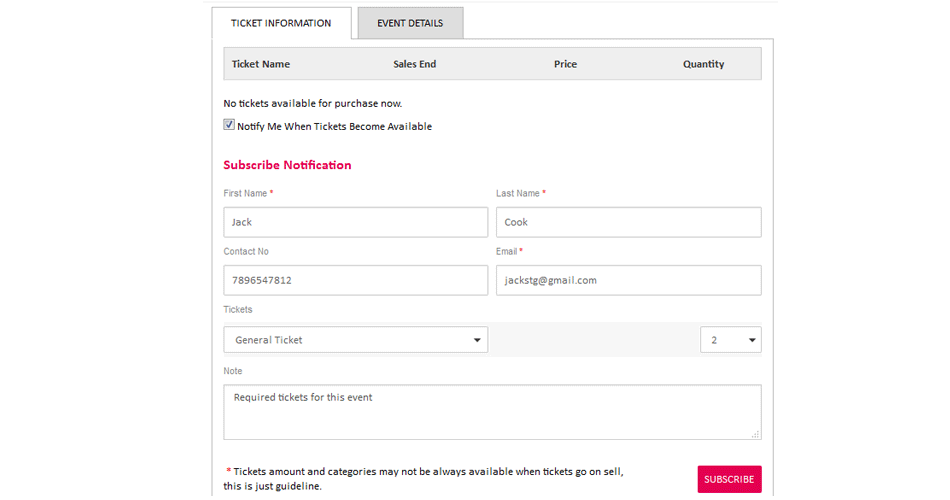The image depicts a form with a clean white background divided into two main sections or tabs, labeled "Ticket Information" and "Event Details," with "Ticket Information" currently selected. This section includes columns for "Ticket Name," "Sales End," "Price," and "Quantity," all written in black text. 

At the bottom of the "Ticket Information" section, a message in pink text states, "Tickets are available for purchase now. Notify me when tickets become available." Next to this message is a checked checkbox labeled "Subscribe Notification." Below this, there is a form field prompting for personal details: 

- First Name: Jack 
- Last Name: [empty]
- Contact Number: 07896547812
- Email: jackstg@gmail.com
- Ticket Type: General Ticket
- Quantity: 2

Further down, there is a note section with the message, "Require tickets for this event." A red star icon highlights the footnote, which reads, "Ticket amount and categories may not always be available when tickets go on sale. This is just a guideline."

In the bottom right corner of the form, there is a prominent red button with white text that reads "Subscribe," indicating the action to finalize the ticket details and notifications preferences.